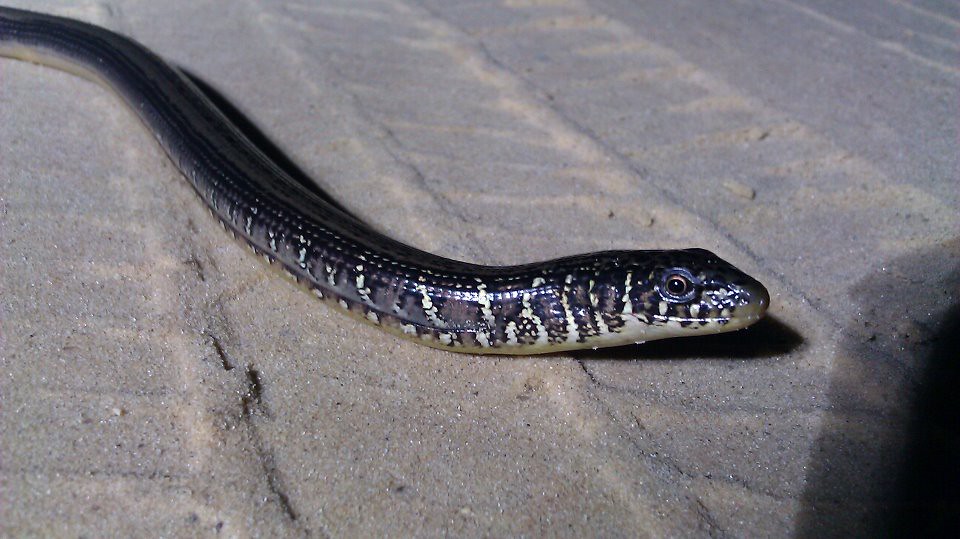In this detailed image, a long snake is seen slithering from left to right across a tan or brown concrete surface, which may also resemble sand. The surface, featuring possible tire tracks or corrugation, adds texture to the background. The absence of reference objects makes estimating the snake's exact size challenging, although its length is evidenced by its extended, sinuous body traversing most of the image. The snake, adorned with distinctive multi-colored markings, displays a dark top, black scales along its dorsal side, and a silver-gray coloring on its flanks, transitioning to a silver underbelly. The snake's black eyes are visibly oriented toward the camera, while its closed mouth maintains a calm demeanor. The snake's unique pattern, resembling tiger stripes or zebra stripes, runs from its head to the tail. A notable shadow occupies the right side of the frame, adding depth and contrast to the scene, while the lighting, potentially natural or from the camera, illuminates the snake's intricate details.